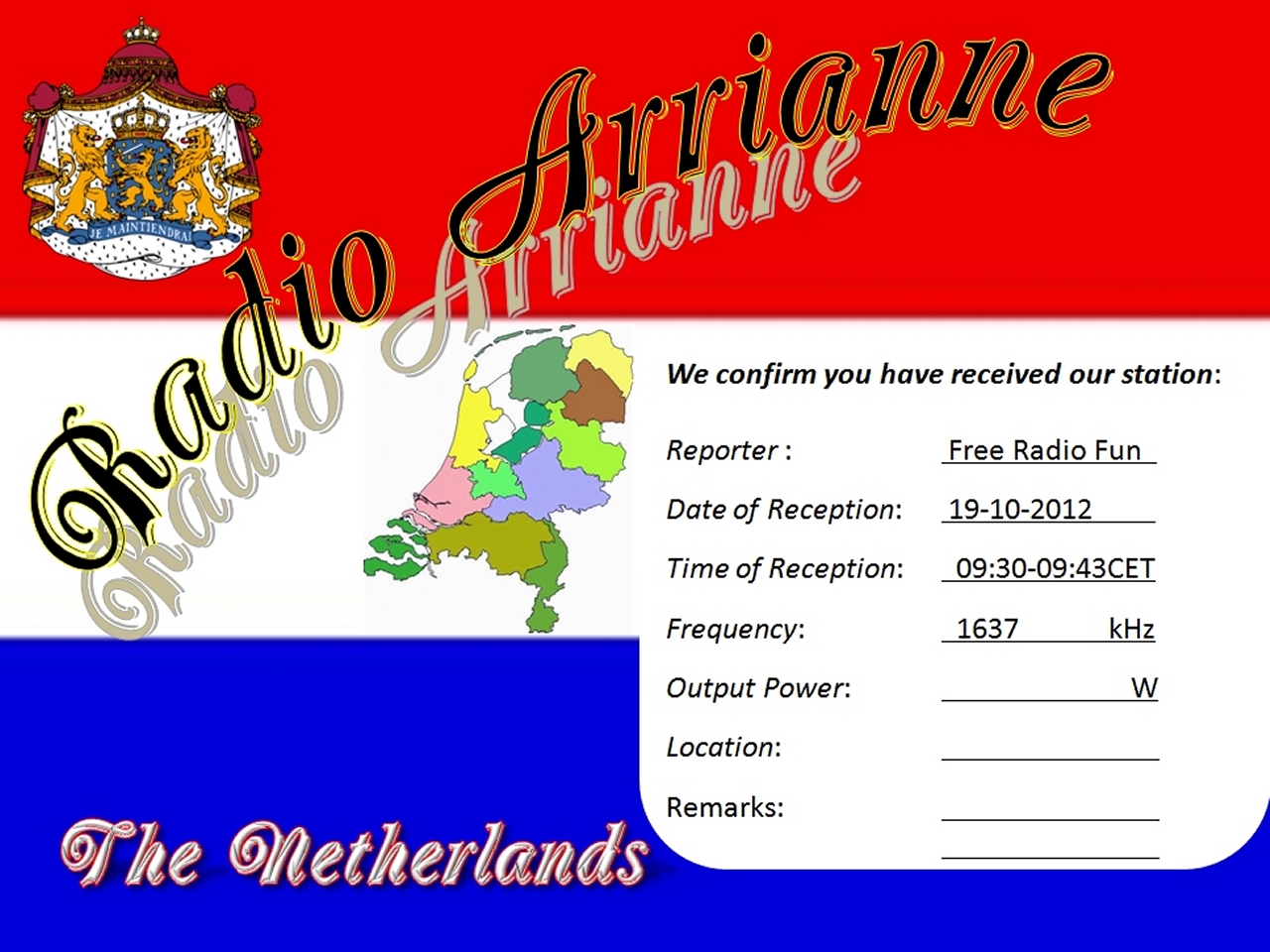The image is a ham radio reception confirmation card, partially filled out, from a group called Radio Ariane. The background of the card features a red band at the top, a white band in the middle, and a blue band at the bottom, resembling a flag. In the upper left corner of the red portion, there's a coat of arms in yellow, red, and blue, featuring text that looks like "Je Maintiendrai" and pictures of lions. In the middle left, extending from the white portion into the red, "Radio Ariane" is printed in black lettering, with a shadow in gray beneath it. Below is a map of the Netherlands in brown, yellow, green, purple, and pink hues. To the right of the map, a white window displays the text, "We confirm you have received our station." Below this text are black lines for details like "Reporter: Free Radio Fun," "Date of reception: 19-10-2012," "Time of reception: 9:30-9:43 CET," "Frequency: 1.637 MHz," and "Output power: W," with the location and remarks fields left blank. At the bottom left of the card, in blue and white lettering, it says "The Netherlands."